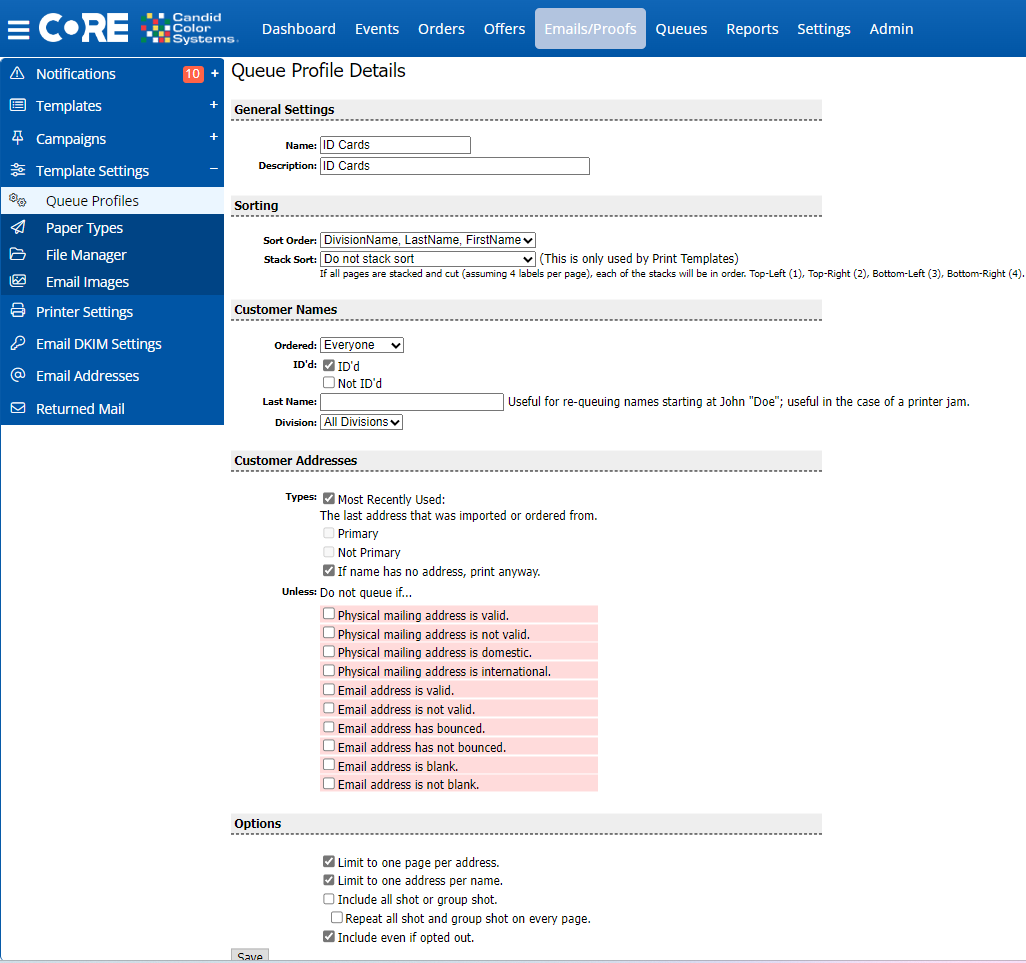A predominantly blue and white webpage features a detailed and structured interface. At the top left, bold white bands frame the text "CORE" in capital letters, with the "O" outlined in dark blue and containing a white circle. Adjacent is a Rubik's Cube-like logo comprising green, yellow, blue, dark blue, white, and red blocks. To its right, the text reads "Candid Keller Systems" in a stacked format.

The bezel at the top contains white-text-on-dark-blue-background clickable buttons, listed as Dashboard, Events, Orders, Offers, and the highlighted Emails/Proofs section, which is in gray and light gray to indicate its selection. Further buttons include Cues, Reports, Settings, and Admin.

The middle section opens with "Cue profile details" in black, followed by a small dark gray rectangle labeled "General Settings" in black text. Below this, two rectangles display: "Names" and "Description," both containing the text "ID Cards."

A subsequent dark gray rectangle, labeled "Sorting" in black text, includes two more rectangles. The first, titled "Sort Area," offers drop-down options for Division Name, Last Name, and First Name. The next, "Stack Short," also provides a drop-down menu, specifying "Do Not Stack Short" and noting in black text that this is used by Print Templates. Detailed instructions follow, describing the stacking order in parentheses.

Another dark gray rectangle is labeled "Customer Names" in black, leading to an area that displays "Ordered" with a drop-down menu currently set to "Everyone." "ID'd" is checked and in gray, while "Not ID'd" remains white. The "Last Name" section suggests its utility for requeuing names, such as "John Doe,” in case of a printer jam. The "Division" drop-down menu defaults to "All Divisions."

Below, "Consumer Address" is encased in a dark gray rectangle. Various buttons mark selections, with "Most Recently Used" and "If Name has no address, print anyway" highlighted. The "Useless" section boldly lists "Do Not Queue If," followed by multiple unchecked options: valid/invalid physical and email addresses, domestic/international addresses, and whether emails have bounced.

A lower gray rectangle labeled "Options" offers several clickable settings, revealing that three of the five visible choices are selected. The "Save" button appears at the bottom left, gray with black text. Selections include "Limit to One Page Per Address," "Limit to One Page Per Name," and "Include Even if Opted Out."

On the left-hand side, a dark blue drop-down menu highlights "Notifications" with a white exclamation-mark triangle and an orange square showing "10+" notifications. Additional options include "Templates," "Campaigns," "Template Settings," "Cue Profiles" (selected, marked with two gears), "Paper Types," "File Manager," and "Email Images" (featuring an image icon). Continuing in dark blue, icons for "Printer Settings," "Email DKM," and "Settings," among others, offer further navigation.

Overall, the webpage is a visually structured amalgamation of functional elements and settings, meticulously crafted for ease of navigation and detailed workflow management.